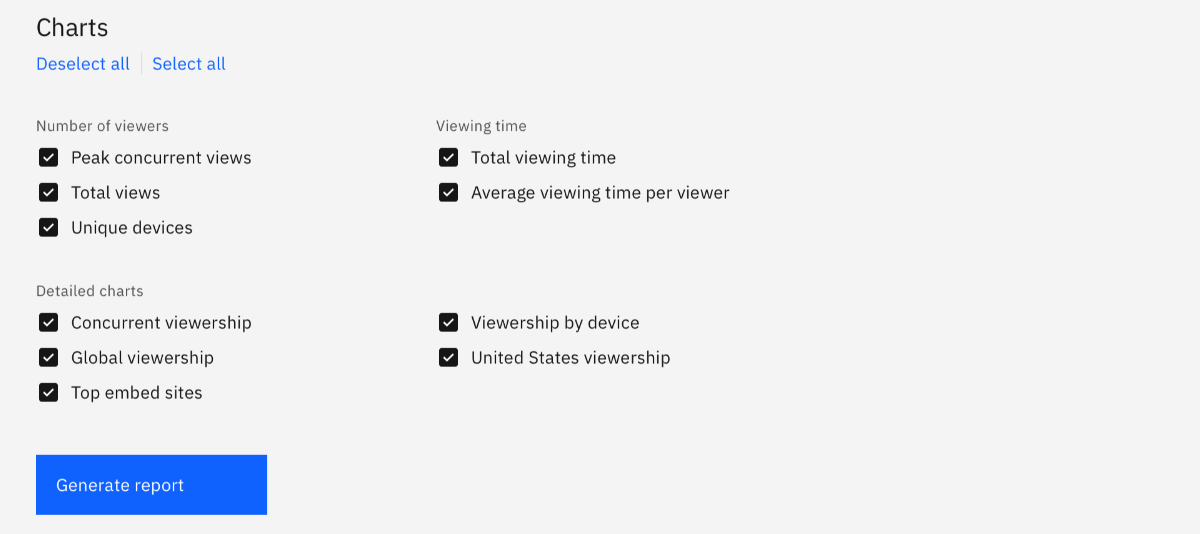This image is a cropped screenshot featuring the charts section of an admin panel on a YouTube analytics page. The background is grey, providing a neutral backdrop to the detailed data display. At the top left corner, "Charts" is prominently labeled in a dark grey font, with a left-pointing arrow adjacent to it, indicating that this section is expanded.

Below the title, there are options for selecting or deselecting various data categories, noted as "Deselect all" and "Select all" in small blue font. The panel displays several main categories and their respective subcategories, each facilitated by checkboxes.

The first main category, "Number of Viewers," is positioned on the left side, and it includes three subcategories: "Peak Concurrent Views," "Total Views," and "Unique Views," all of which are checked.

Moving down, the "Detailed Charts" category appears towards the bottom left, featuring three options: "Concurrent Viewership," "Global Viewership," and "Top Embed Sites," each selected as well.

To the right side, the "Viewing Time" category lists two subcategories: "Total Viewing Time" and "Average Viewing Time per Viewer," both of which are also checked.

At the bottom right, there are two additional options: "Viewership by Device" and "United States Viewership," which are both selected.

In the bottom left corner lies a blue button labeled "Generate Report" in white font, ready to compile the selected data into a comprehensive report. The remaining portions of the page are cropped out.